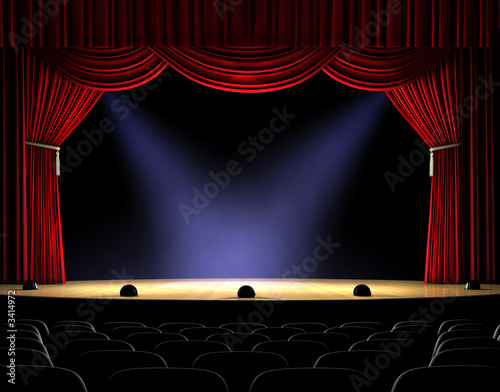The image depicts a vintage, old-fashioned theater stage from the audience's perspective. Dominated by an elegant red velvet curtain with tasseled, silver tiebacks, the stage gives off a grand and historical vibe. This curtain frames a rectangular blue backdrop, illuminated by two white rays of light that form a V-shape from the top corners to the stage's center. The floor of the stage is a warm yellow, showcasing five dome-shaped items—possibly lights or speakers—lining the edge. Visible at both the top and side of the stage is an Adobe Stock watermark, including the text “Adobe Stock” with the number 3414972, which confirms the imagery's sourced nature. The theater is empty, with rows of black, vacant seats in the foreground. The overall image appears more like an artistic illustration or painting, rather than a photograph, highlighting a serene yet anticipatory ambiance, as if ready for a ballet or modern dance performance.